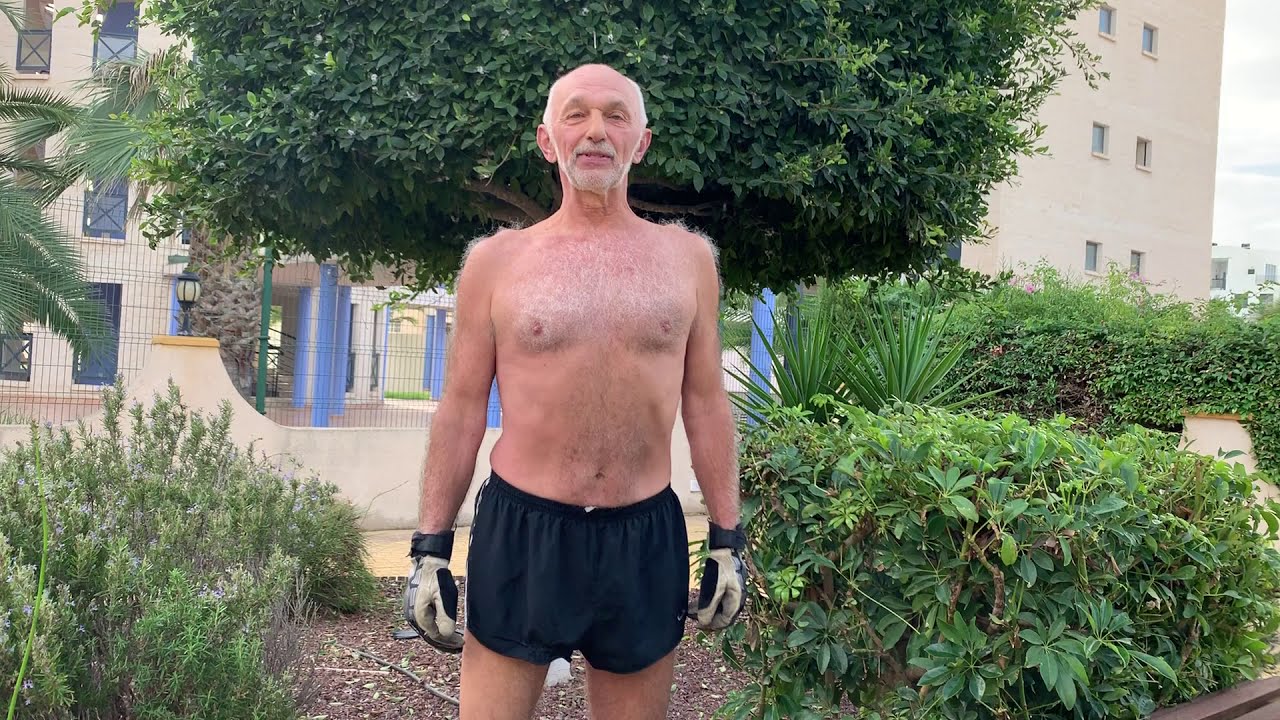In this detailed outdoor photograph, an elderly, physically fit man in his 60s or 70s stands confidently in front of an apartment building. He is shirtless and wears only a pair of black shorts and gray gloves, suggesting he might be engaged in some yard work. His bald head is complemented by a gray beard and mustache, and grayish-white hair is visible on his chest and shoulders. The man stands between vibrant green bushes, with a lush tree just behind him. The tree's full green leaves obscure the trunk, adding a natural frame to the scene. Behind the tree, a gray, multi-story apartment building with blue pillars rises in the background. The sky overhead is gray, adding a neutral tone to the vivid greenery. The man appears to be in conversation with the photographer, giving the image a personal and engaging feel.